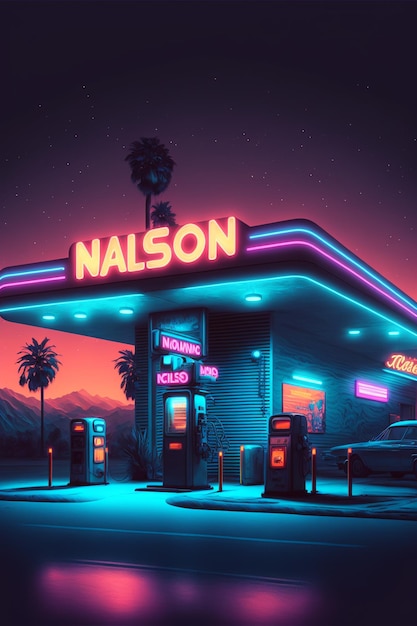This captivating painting portrays a neon-lit service station set against a twilight backdrop, where a dark starry sky transitions into a gradient of pink, orange, and peach hues, reflecting the setting sun. The awning of the station prominently features the name "NALSON" in large, illuminated yellow neon letters, surrounded by blue and pink neon tubes that accentuate the building's roofline. Below, the awning casts an ethereal glow, highlighting a small booth and three gas pumps with orange indicator lights, signifying they are active. A solitary car is parked to the left of these pumps, nestled under the overhang. In the distance, palm trees silhouetted against the vibrant sky add a tropical touch, with mountains faintly visible beyond. The gas station itself is adorned with various neon signs, including some in cursive text, which are partially obscured but contribute to the overall ambiance. The soft, airbrushed tones of purple, blue, and peach blend seamlessly, creating an enchanting and surreal scene that seems almost dreamlike, fusing vivid neon lights with a muted yet mesmerizing aesthetic.